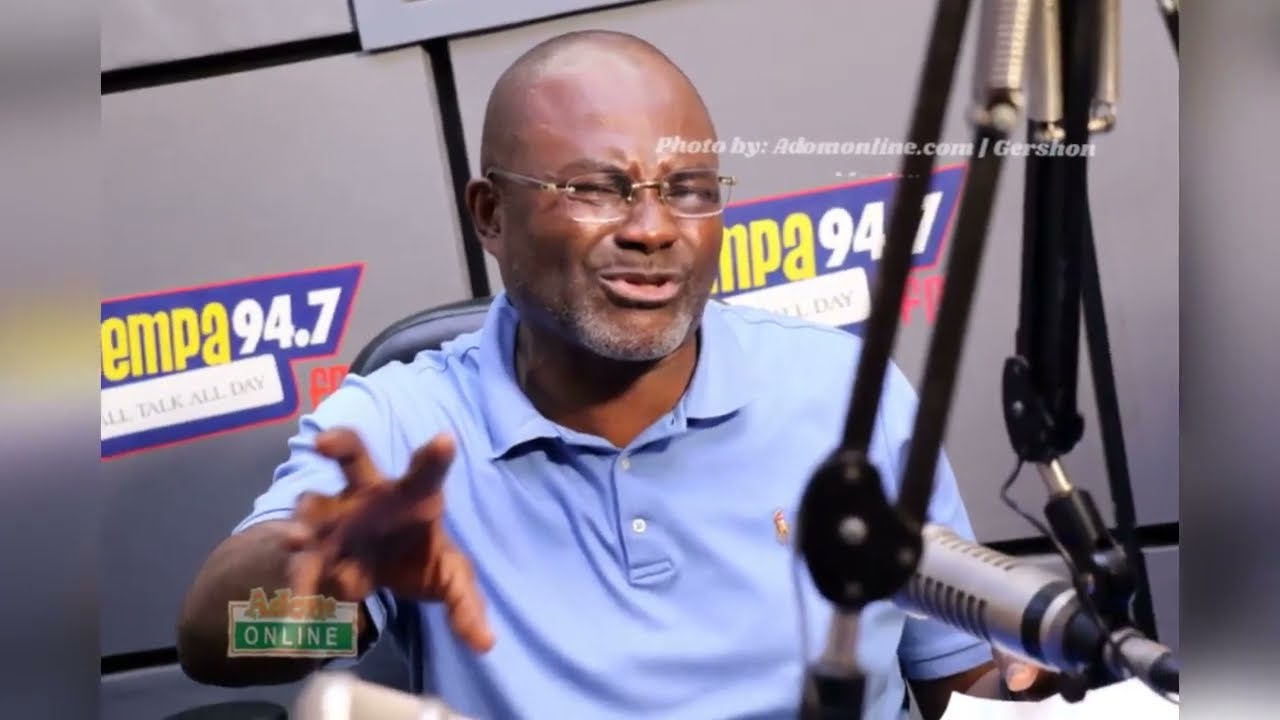The image captures an African American man seated in a radio studio, actively engaged in speaking into a prominently displayed, large gray radio microphone mounted on a flexible black arm. The man, who has dark skin, a bald head, and a short grayish goatee, is wearing rimless glasses and a light blue, collared, short-sleeved shirt. He seems to be in the middle of a speech, with his lips forming a word and his right hand gesturing expressively. His intent expression suggests he is deeply focused on his broadcast. Behind him, the studio's gray wall features the radio station's logo, "EMPA 94.7," with "EMPA" in yellow letters and "94.7" in white, accompanied by a blue background and red border. Next to the logo, white text reads "photo by adamonline.com/Gershon." Additionally, several identical stickers stating "Tempo 94.7, All Talk All Day" are visible in the vicinity. The radio studio setting is further confirmed by various objects like boxes or file cabinets in the background.